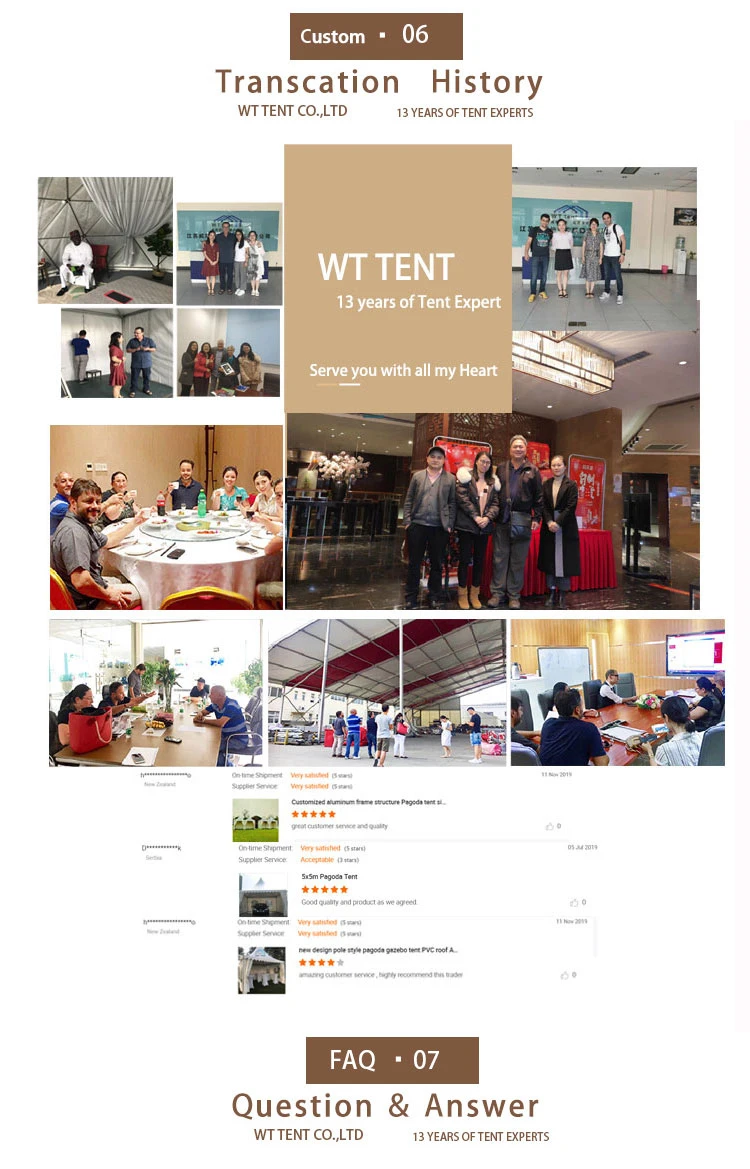In this image, we see a detailed display of a company's tent offerings and customer feedback. The image prominently features a "Customized Aluminum Frame Structure Pagoda Tent" provided by Tent Experts, a company with 13 years of experience in the industry. The tent dimensions are specified as 5 by 5 meters, and the product boasts high-quality materials, particularly a PVC roof with a new design pole style.

Customer reviews and ratings are also highlighted, showcasing a five-star review that praises the company for great customer service and product quality, mentioning "very satisfied." Another review gives a three-star rating, labeled as "acceptable." A final review awards the newly designed Pagoda Tent four out of five stars, complimenting the amazing customer service.

Key details and codes such as "custom 06," "transaction history," and "WC10 code" are indicated, although WC10 appears limited. This text adds a layer of authenticity and context, reinforcing the company's commitment to serving customers with all their heart over their extensive period of operation.